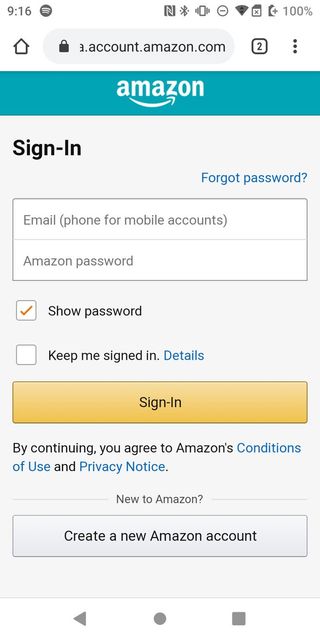A detailed screenshot of an Amazon sign-in page displayed on a smartphone. The time reads 9:16, and there is a recognizable Spotify logo next to the clock. Along the top right, several icons are visible, including those indicating Bluetooth, vibration mode, Wi-Fi connection, signal strength, and a 100% battery level. The URL displayed is account.amazon.com, with two browser tabs open. To the left is a home button, and on the far right are three vertically stacked dots, commonly used to signify additional options. 

The blue header bar prominently features the white Amazon logo, and below it, the text "Sign-In" appears in large, bold lettering. Options such as "Forget Password" and a text link to recall the password if forgotten are present. The sign-in fields include placeholders for "Email or mobile phone number" and "Amazon password," each enclosed in thin gray rectangles. 

Below these fields, there are two checkboxes. The first checkbox, next to the gold "Show password" option, is checked, while the second checkbox, labeled "Keep me signed in," remains unchecked. At the bottom of the form is a gold-colored button labeled "Sign-In." Beneath this button, a message states, "By continuing, you agree to Amazon's Conditions of Use and Privacy Notice." Additionally, there's an option for new users to create an Amazon account, labeled "New to Amazon? Create a new Amazon account."

The navigation menu is visible at the bottom of the screen, providing easy access to other features.